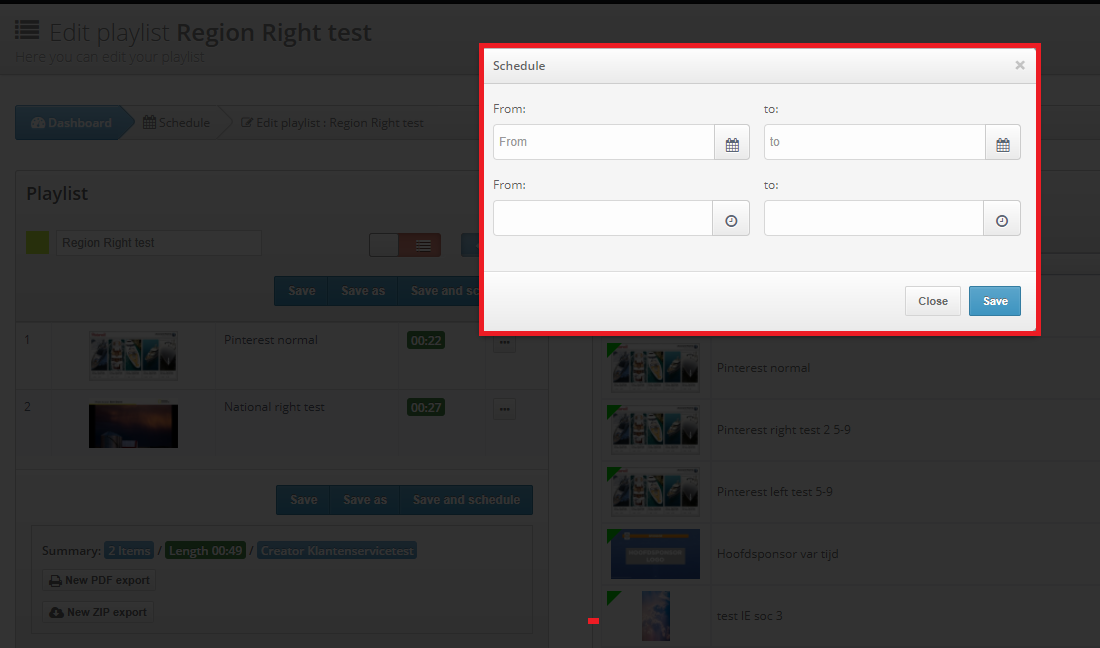The image depicts a webpage with a gray overlay that gives it a subdued, shadowed appearance, making the content somewhat difficult to discern. The central content of the webpage appears to be a playlist section designated for a "region rate test," prominently featuring what seem to be album or song covers, though the details of these images are not clear.

On the right-hand side, there is a vertical list, likely associated with Pinterest, displaying several thumbnail images or covers that are presumably linked to pins on the platform.

In the middle of the screen, a pop-up box with a light gray and white background and a hot pink border is visible. The pop-up is labeled "Schedule" at the top in light gray text, accompanied by a close button (X) at the top-right corner. Inside the pop-up, there are two pairs of "From" and "To" fields presumably for setting a schedule or time range. At the bottom right corner of the pop-up is a blue "Save" button, which allows the user to save their inputted information.